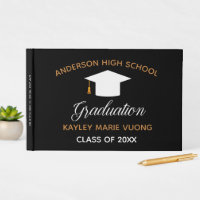This image features a small square photograph showcasing a white background. Dominating the center of the composition is a black rectangular graduation booklet standing upright on a white surface. The booklet is adorned with dark brown lettering at the top that reads "Anderson High School." Beneath this arching text, a white silhouette of a graduation cap with a gold tassel hanging from the left side adds a celebratory touch. In a graceful white script, the word "Graduation" is elegantly displayed below the cap. Further down, in prominent brown capital letters, the name "Kaylee Marie Vuong" is inscribed. The bottom section reads "Class of 20XX" in white capital letters. A gold ballpoint pen lies in front of the booklet, positioned towards the lower right of the image, while a small green succulent in a round cream-colored planter appears partially on the left. The meticulous arrangement and choice of colors create a harmonious and formal presentation, capturing the essence of a meaningful graduation memento.